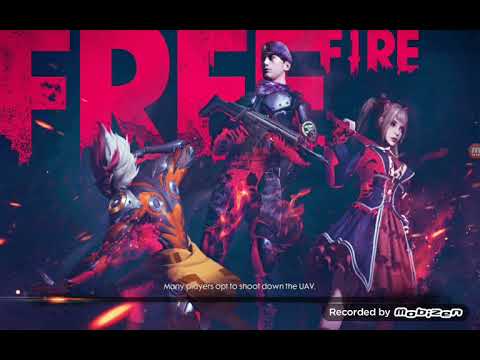The image is the opening screen of a video game, presumably called Free Fire, as indicated by the prominent text in bold red letters reading "Free" and smaller red letters "Fire." The background is entirely black, highlighting the three characters positioned in the foreground. 

In the center stands a male character dressed in military-style armor. This character is holding a large rifle and has some type of headgear. His pants seem to have flames on them, contributing to the red and orange hues in his outfit. To the right, a young female character is dressed in a checkered dress with red and black frills. She sports pigtails with brown hair and is holding an item, possibly a sword or a bat, over her shoulder. The last character on the left appears to be a muscular martial artist wearing orange and black armor with red accents. This character is also donning a mask that resembles a fox or wolf, giving an impression of mystery as he's cloaked in shadow.

The screen also features a loading bar at the bottom, accompanied by the text "many players opt to shoot down the UAV," hinting at gameplay elements. Additionally, there's a small text in the bottom right corner that reads "recorded by Mobizen" on a white background, indicating the method of screen capture. Visually, the characters have an anime or cartoonish style, complementing the overall dynamic and action-packed theme of the game's introduction screen.